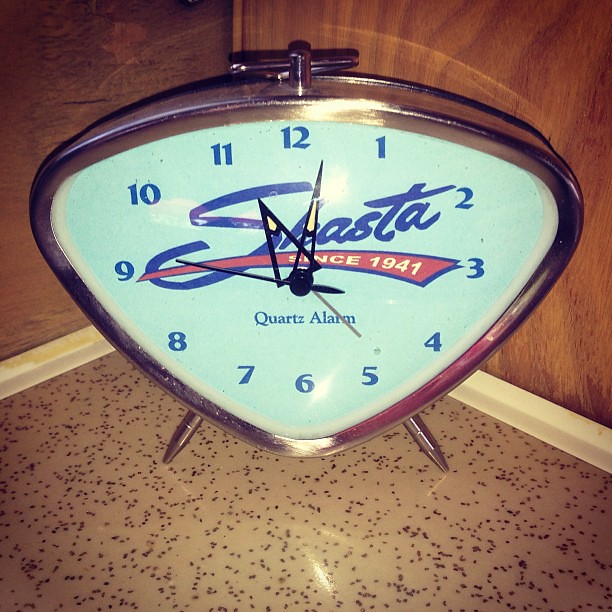This image depicts an antique wind-up clock sitting on the floor in the corner of a room. The clock’s unique shape resembles a softly curved triangle with rounded edges. It features a silver metallic housing and rests on two small, pointed chrome feet. The room's walls are made of wood, while the floor is a speckled tile, predominantly beige with black flecks, and bordered by a thin white baseboard.

The clock itself showcases a white face encircled by a metallic lining. The numbers on the clock are a distinct dark blue, complemented by arrow-shaped hands that are outlined with yellow tips. A prominent feature on the clock's face is an inscription reading "Shasta since 1941" in blue lettering, with "since 1941" underlined in red with white font. Below this, the words "Quarks Alarm" are printed in blue. There is also a small silver gear on top of the clock, used for winding, indicative of its vintage mechanical design. The current time is displayed as shortly after 11 o'clock.